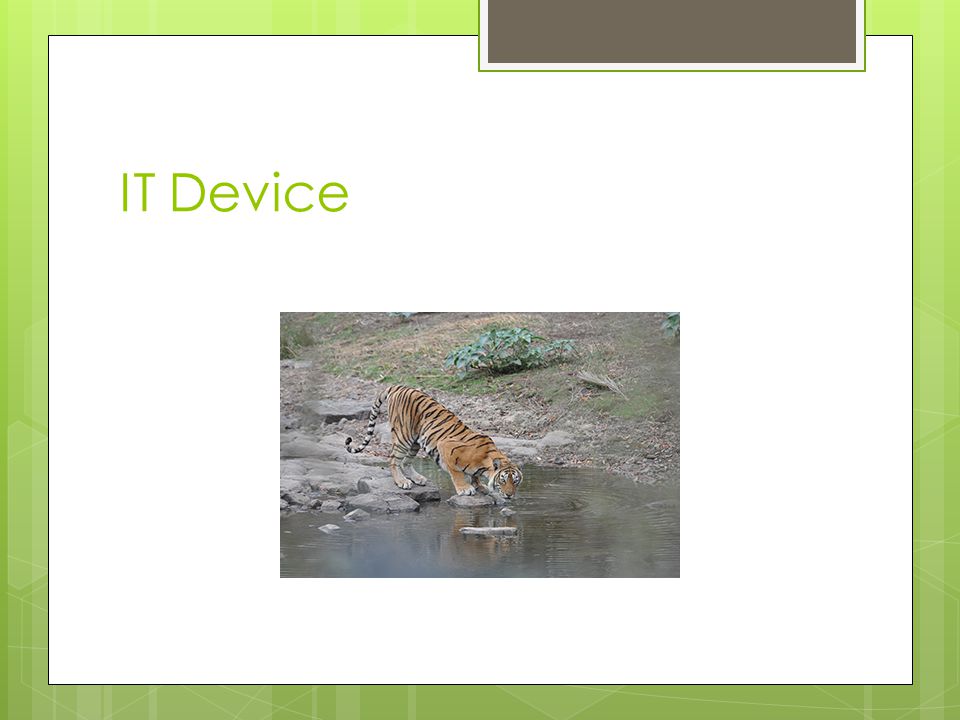This image appears to be a slide from a presentation featuring a white background with a gradient green border that transitions from a light green at the top to a sage green at the bottom. Subtle design details can be discerned within this green border. On the top right-hand side within the border, there is a brownish-colored box surrounded by a white edge. Dominating the central part of the slide is the text "IT DEVICE" in light green letters that match the border. Below this text, there is a photograph of a tiger, characterized by its orange fur and black stripes, drinking from a stream or pond. The tiger's front paws are partially submerged in the water, while its back paws rest on nearby rocks. The scene includes some vegetation—including grass, small plants, and hints of flowers—confined to a rocky and slightly dirt-covered background. The tiger is positioned centrally within the image, amplifying its prominence against the outdoor setting encapsulated on this slide.